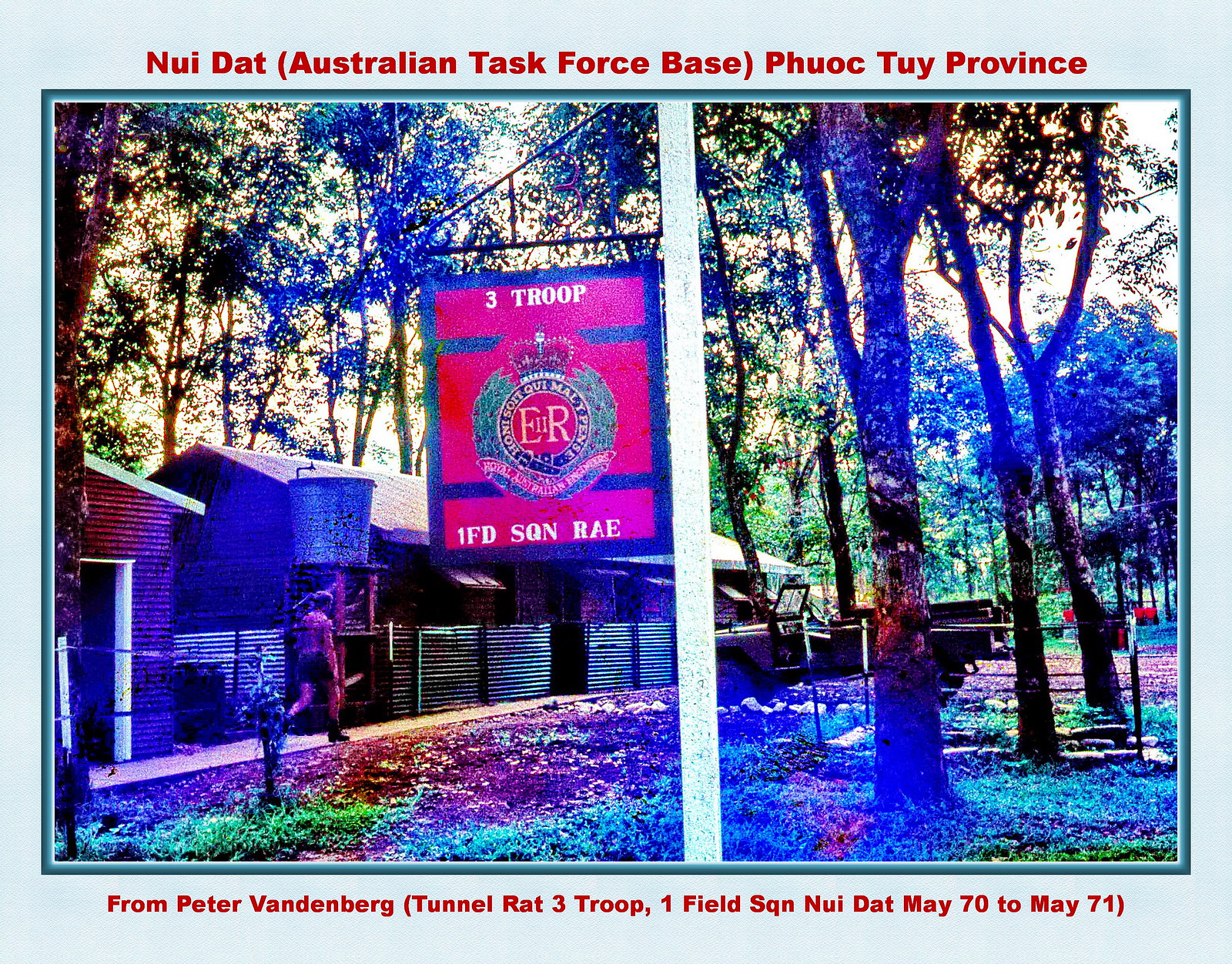This is a detailed, descriptive caption for a Vietnam-era photograph taken at NUI DAT, Australian Task Force Base, Phuoc Tuy Province. The picture showcases a heavily wooded area with several brown, semi-metallic barracks that may have tin roofs. In the foreground, an olive-green military jeep without a top is parked on a light wooden sidewalk. A single man dressed in a t-shirt and shorts is walking down this sidewalk. Dominating the center of the image is a tall white pole with a red square sign that reads "3 Troop, ER, 1 FD, SQN, RAE." The sky appears partly cloudy, complemented by the soft pink, blue, and white hues that dominate the photograph, though the resolution is not very high. Surrounding the scene is a darker shade of blue border. At the top of the entire image, the text in red reads "NUIDAT, Australian Task Force Base, Phuoc Tuy Province," and at the bottom, it states, "From Peter Vandenberg, Tunnel Rat 3 Troop, 1 Field SQN, NUIDAT, May 70 to May 71."